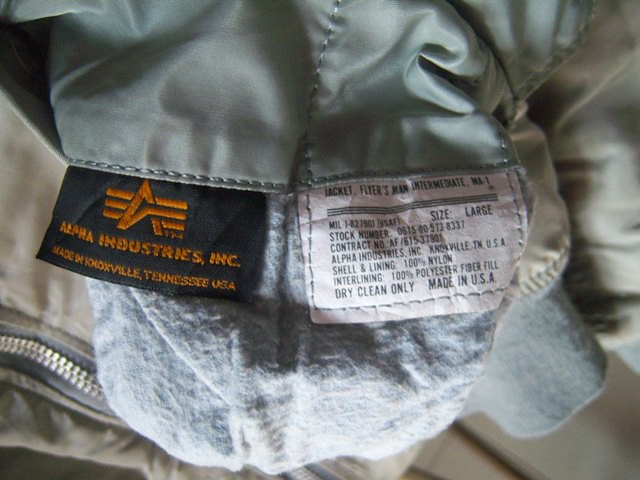The image depicts a close-up of a jacket, primarily light greyish-green in color, made by Alpha Industries Incorporated in Knoxville, Tennessee, USA. The jacket features a front zipper and elastic cuffs at the wrists. The focal point of the image is two labels sewn into the jacket. One label is black with orange detailing, displaying the logo of three horizontal bars and an 'A' shape, along with the text "Alpha Industries Inc." and "Made in Knoxville, Tennessee, USA." The other label is white with black text, indicating it as a "jacket, flyers man's intermediate." This label also lists the stock number, contract number, shell and lining material as 100% nylon, interlining as 100% polyester fiberfill, and specifies "dry clean only" along with "Made in the USA." The stitching on both labels matches the jacket's material color.